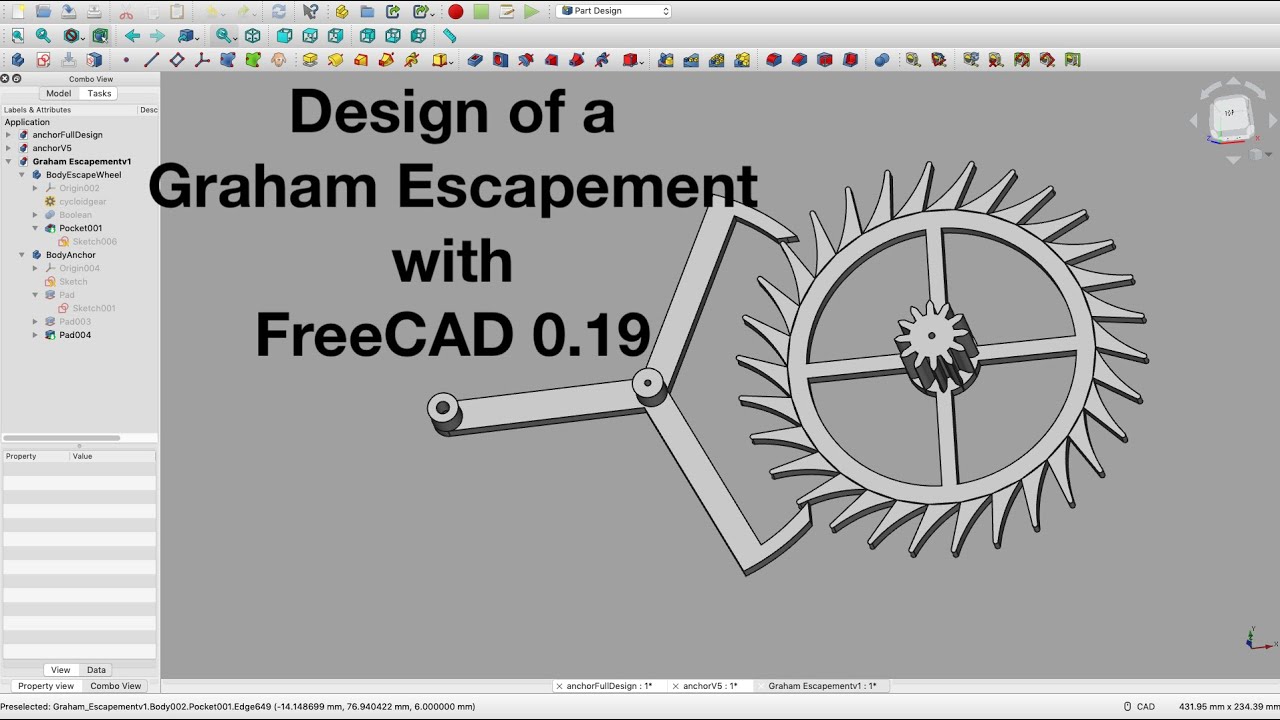The image is a screenshot of a web page showing a computer monitor with a design program, likely FreeCAD 0.19, being used to design a "Greyhound Escapement." Dominating the screen is a detailed 3D CAD drawing featuring a circular gear with numerous pointed teeth along its outer edge, forming a complex structure of cross beams inside. At its center is a smaller gear, which appears connected or welded in place. To the left of this gear, a metallic arm-like structure extends outward, resembling a claw with two handles, one on the top and one on the bottom, and a horizontal handle on the left. This arm or clamp interacts with the wheel, suggesting a mechanical function. The software interface is predominantly in shades of gray and white, with an array of icons displayed along the top and left sides, while the bottom of the screen contains file details. In the top right corner, a small icon offers 3D rotation capabilities, providing the user a preview area with arrows for manipulating the design in three-dimensional space.